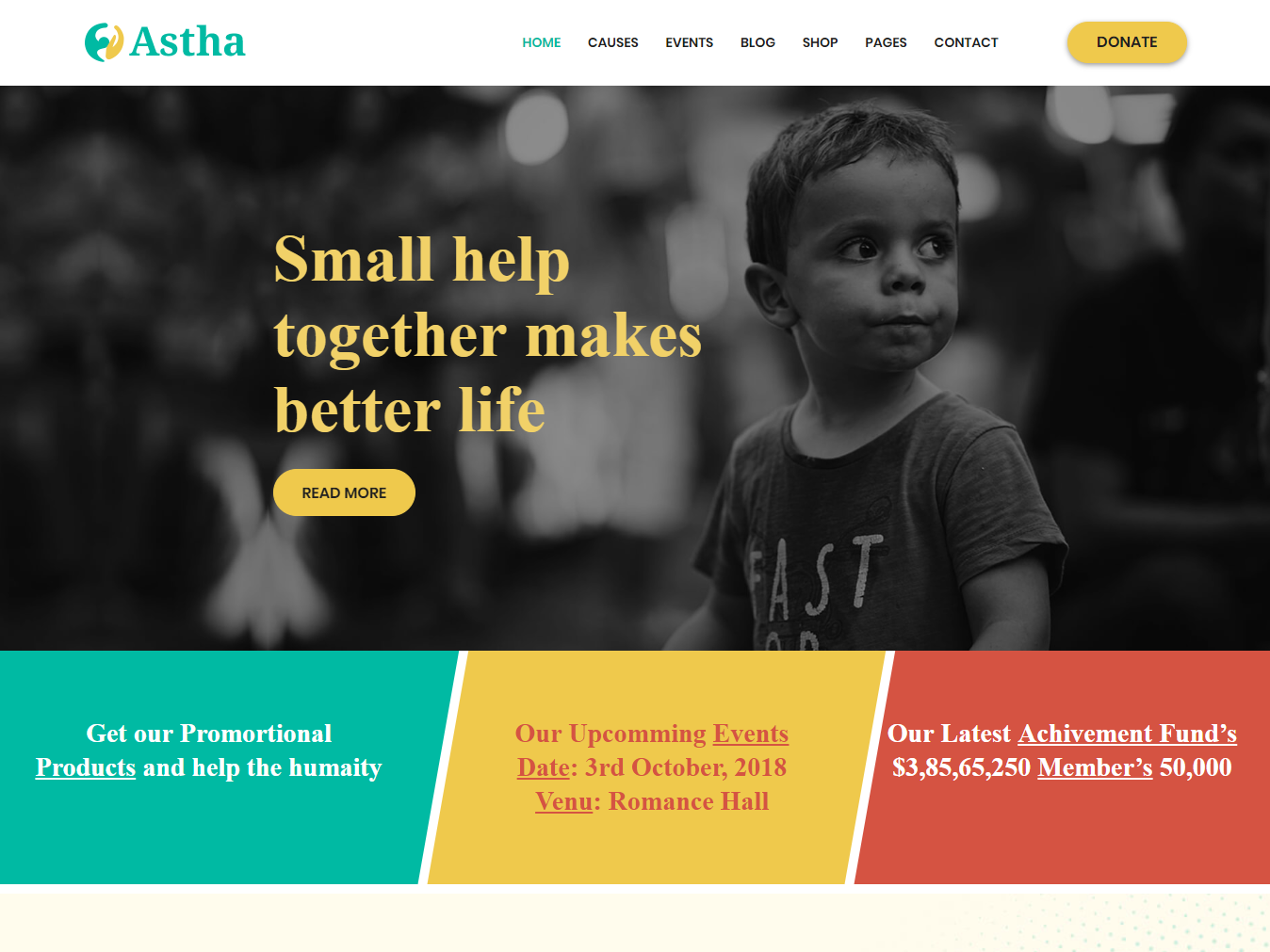The image features a colorful and detailed layout designed to promote a charitable organization. In the top left corner, there's a green and gold symbol accompanied by the word "ASTHA" in bold letters. To the right, a navigation menu includes options such as Home, Causes, Events, Blog, Shop, Pages, and Contact. Nearby, a prominent yellow button labeled "Donate" stands out.

Centered in the image is a poignant black and white photograph of a young boy, overlaid with the text, "Small help together makes a better life." Below this, another yellow button invites viewers to "Read More."

Further down, a teal-colored box urges support, stating, "Get our promotional products and help the Humeichi," albeit with notable misspellings. To the right, a yellow box announces an upcoming event scheduled for October 3, 2018, at Romance Hall.

Lastly, a red box highlights a recent achievement, detailing that a fund reached 38,565, with 250 members contributing to a 50,000 goal.